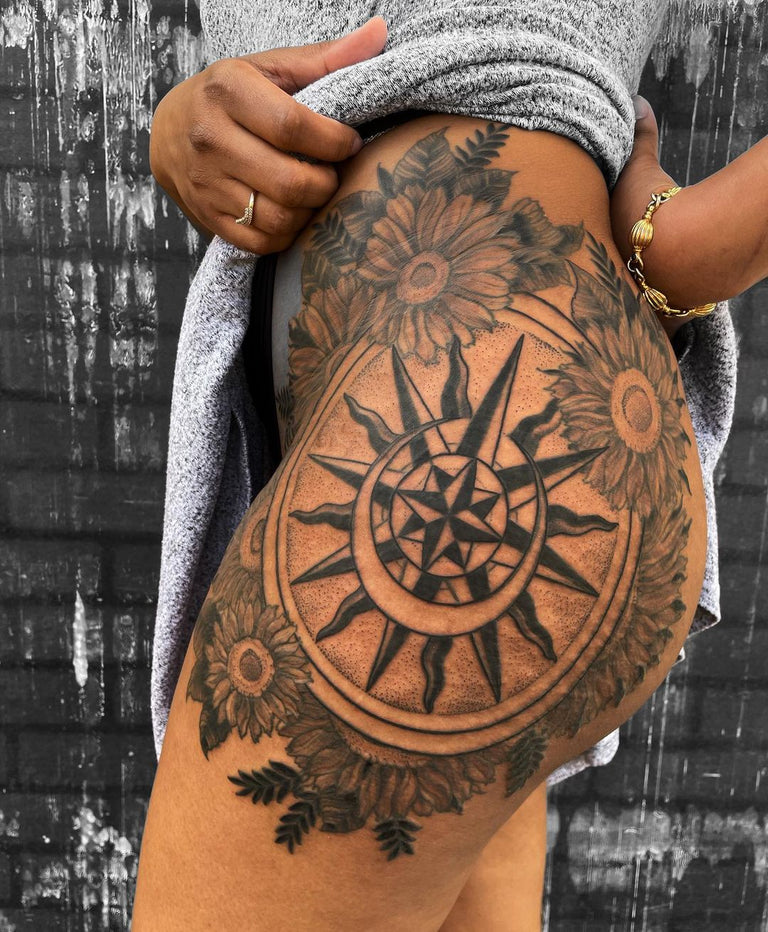A richly detailed image captures a side profile of a woman exhibiting her newly completed tattoo on her left thigh and waist. Her darker skin tone suggests she may be African American or Latino. The visible section of her body extends from her lower torso to her thigh, and her face is not shown. She is standing before a gray brick wall that features white paint running down its surface. The intricate black and white tattoo spans from her lower torso down to her thigh, with a prominent compass at the center flanked by daisy and sunflower designs that travel upwards toward her hip. She has pulled up her gray clothing, likely a shirt or dress, to fully display the elaborate tattoo. Additionally, she is adorned with some jewelry, including a golden bracelet and a ring on her finger, distinctively contributing to the composition of the scene.